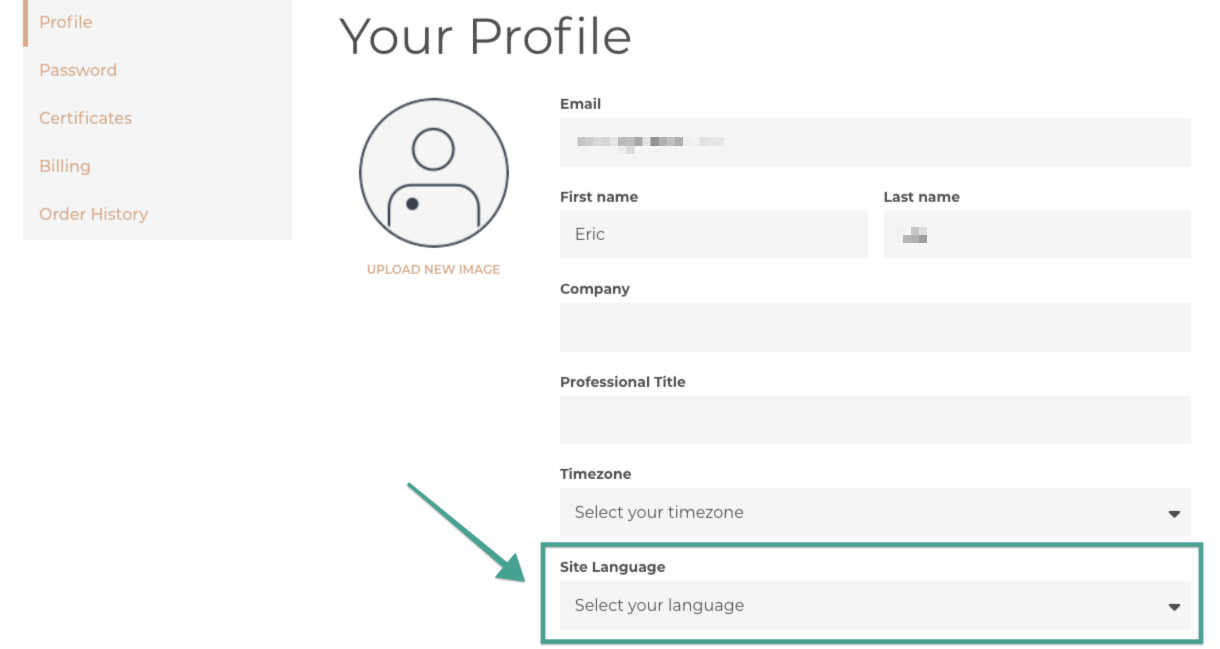**Detailed Profile Page Screenshot Caption:**

The image is a detailed screenshot of a profile page. On the extreme left side of the page, there is a narrow, vertical menu with five tabbed options, arranged from top to bottom as follows: Profile, Password, Certificates, Billing, and Order History. Each of these tabs is housed within a small rectangular section.

The main section of the page displays the "Your Profile" tab, where users can input and modify their personal information. Fields available for editing include: Email, First Name, Last Name, Company Name, Professional Title, Time Zone, and Site Language. Notably, the email field has been pixelated for privacy reasons. 

The Site Language field is highlighted with a turquoise-colored rectangle, accompanied by an arrow pointing to it, drawing attention to this specific input section. The prompt within the Site Language dropdown menu reads, "Select your language." Similarly, the Time Zone field also employs a dropdown menu for selection.

At the top of the main page, beneath the heading "Your Profile," there is a circular avatar placeholder displaying an outline of a head and shoulders. Users are encouraged to upload a new image in this space, with a prompt written in peach-colored text reading "Upload new image." This UI element ensures users can personalize their profile with a photo of their choice.